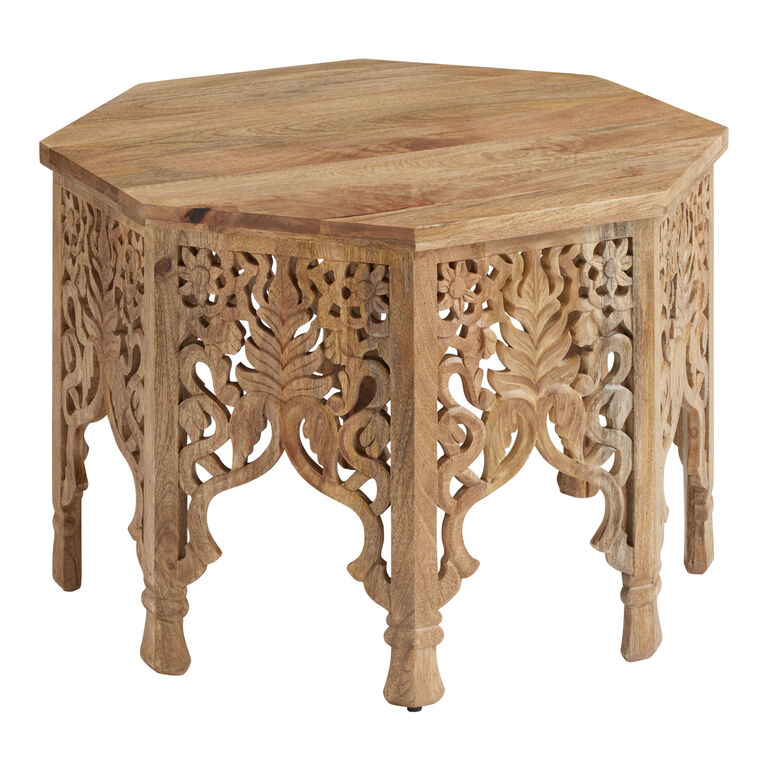This image showcases a highly ornate wooden table set against a completely white background. The table's top is octagonal and crafted from a light-colored, rough wood that lacks any glossy finish. Each of the table's eight legs features intricate floral carvings, embellished with patterns of leaves and vines that cascade halfway down the legs. The carvings include cutouts that allow the white background to peek through, enhancing the decorative effect. Additional detailing is found at the bottom of each leg, where they flare out slightly and include protective elements. The table, potentially of Indian or Asian craftsmanship, appears handmade and well-preserved, devoid of any visible damage, and represents a fine example of antique woodworking skill.